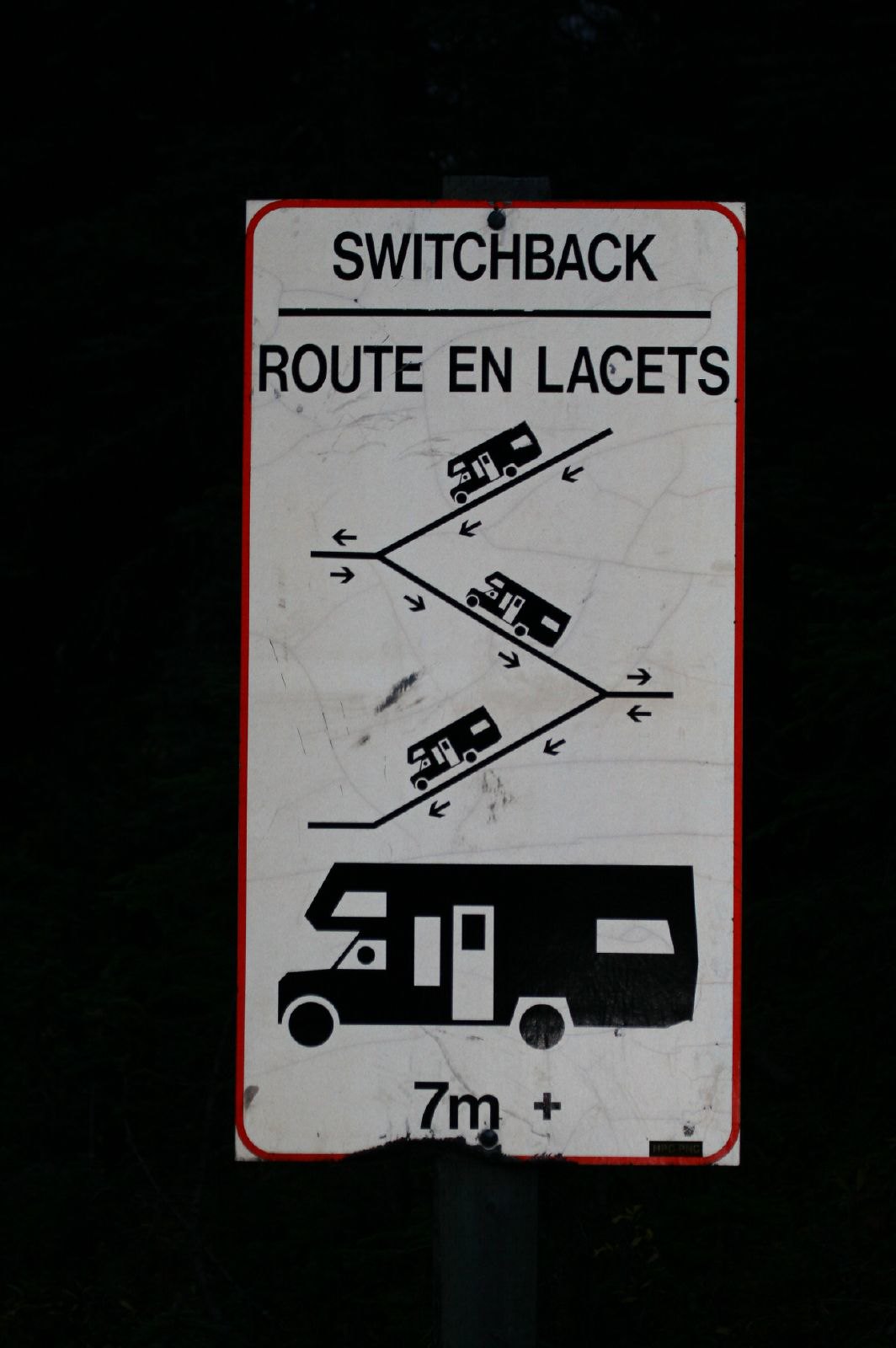The image captures a photograph taken outdoors, likely at night, featuring a sign with a black background and detailed visuals. The focal point is a white rectangular sign, approximately an inch and a half wide and three inches tall, mounted on a gray pole with a red outline trimmed with beveled corners. The sign is held in place by bolts visible at the top center and bottom center.

At the top of the sign, "Switchback" is written in black print, underlined, and set against the white background. Below it, "Route en Lacets" is displayed, again in black text. A detailed diagram occupies the majority of the sign, illustrating the route of what appears to be RVs navigating a winding road. The road slopes from the upper right to the lower left, with a small RV descending and arrows indicating the direction. The road levels out in the center but continues with multiple segments, showing arrows pointing in various directions to depict the complex route. Another RV is illustrated moving upwards against the direction of the arrows on one slope, adding to the intricacy of the scene.

At the very bottom of the sign, a black silhouette of a larger RV is positioned above the text "7M+" indicating a distance or a requirement. The entire sign contrasts sharply against the dark background, suggesting the photo was taken at night.